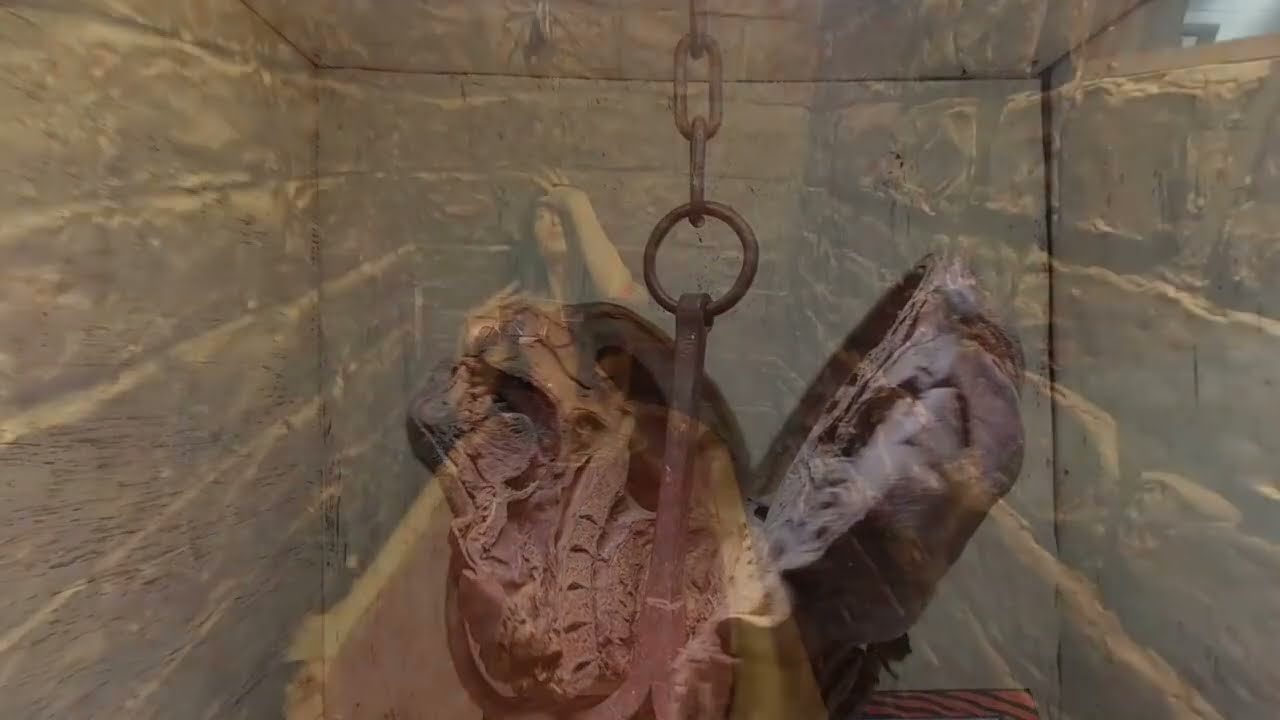This intriguing and somewhat eerie image appears to be taken inside a small, stone-walled room with rough-textured, white-painted bricks. Dominating the center of the photograph is a dark brown metal chain that hangs from the ceiling, culminating in several hooks. These hooks seem to hold what could be either a rock, a fossil of a dinosaur head, or disturbingly, a human skull split open at the center, revealing its inner structure.

A glass pane appears to be in front of this display, adding a layer of reflection to the image. The reflection shows a woman with Caucasian skin tone and long, dark brown hair, seemingly behind the camera. Her head is tilted slightly back, and her left hand is raised, covering part of her forehead with her fingers splayed open. This woman could also be holding the camera, as suggested by the reflection. She is wearing a ring on the middle finger of her left hand. The overall color palette of the image is predominantly tan and brown, contributing to its mysterious and unsettling atmosphere.